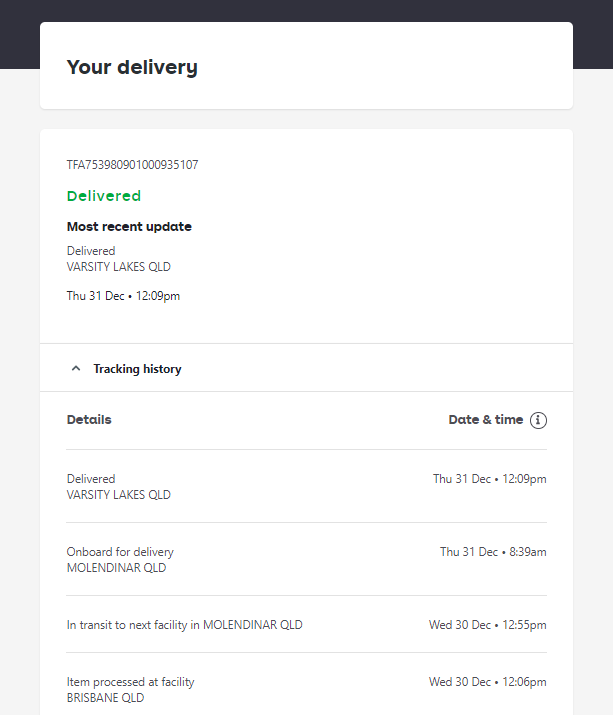The image shows a delivery status update from an app. At the top, a white rectangular box features the text "Your Delivery" in black. Below this, in a large white box, there is a tracking number: "TFA-753-980-90-1000-935-107." Underneath the tracking number, the word "Delivered" is prominently displayed in green, followed by "Most Recent Update" in bold black font. The most recent update location is shown as "VARSITY LAKES QLD."

Following this, the date and time of delivery are provided: "Thursday, 31st of December, 12:09 p.m." The caption then includes sections labeled "Tracking History" and "Details" with corresponding columns for "Date and Time." The detailed tracking history lists the following:

1. "Delivered" at "VARSITY LAKES QLD" on "Thursday, December 31st, 12:09 p.m."
2. "On board for delivery" from "Mullender QLD" on "Thursday, 31st of December, 8:39 a.m."
3. "In transit to next facility" from "Mullender QLD" on "Wednesday, December 30th, 12:55 p.m."
4. "Item processed at facility" in "Brisbane QLD" on "Wednesday, December 30th, 12:06 p.m."

This detailed tracking information encapsulates the journey of the delivery from initial processing to the final delivery at Varsity Lakes QLD.